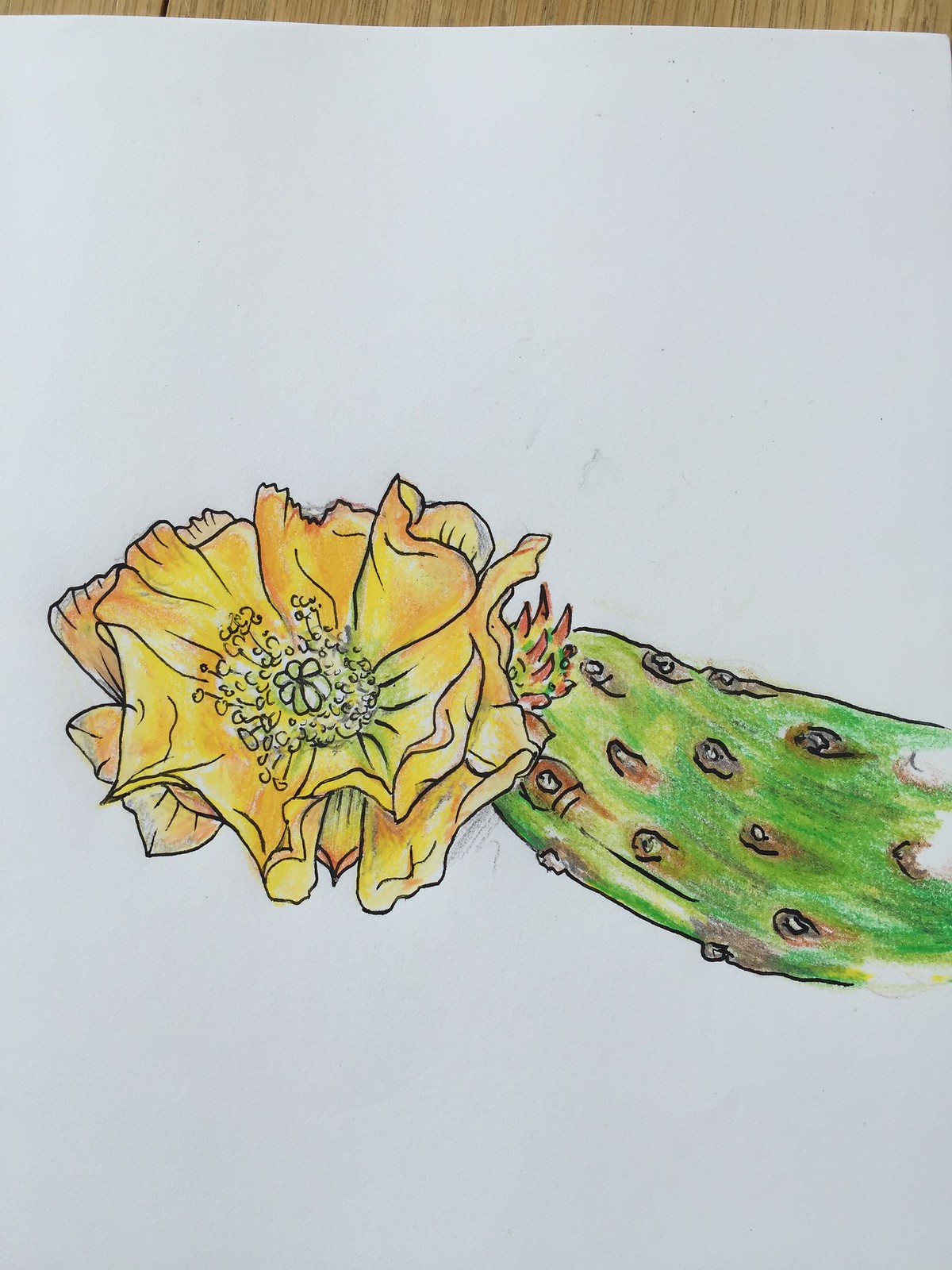The image features a hand-drawn depiction of a fully blossomed, large yellow flower with orange tips, intricately detailed and possibly colored with markers. The flower takes center stage on a white piece of paper, which lies atop what seems to be a wooden table. The bloom reveals layers of petals with a mix of yellow and orange shading for dimension, and an inner arrangement that includes a smaller white flower and black-drawn leaves. Attached to or positioned near the flower is a green, cacti-like structure with ridges and small pink nodules, adding a textured contrast to the composition. The overall effect is a vibrant, artistic rendering that combines digital and hand-drawing techniques, emphasizing the vibrant coloration and detail of the flower and its surroundings.